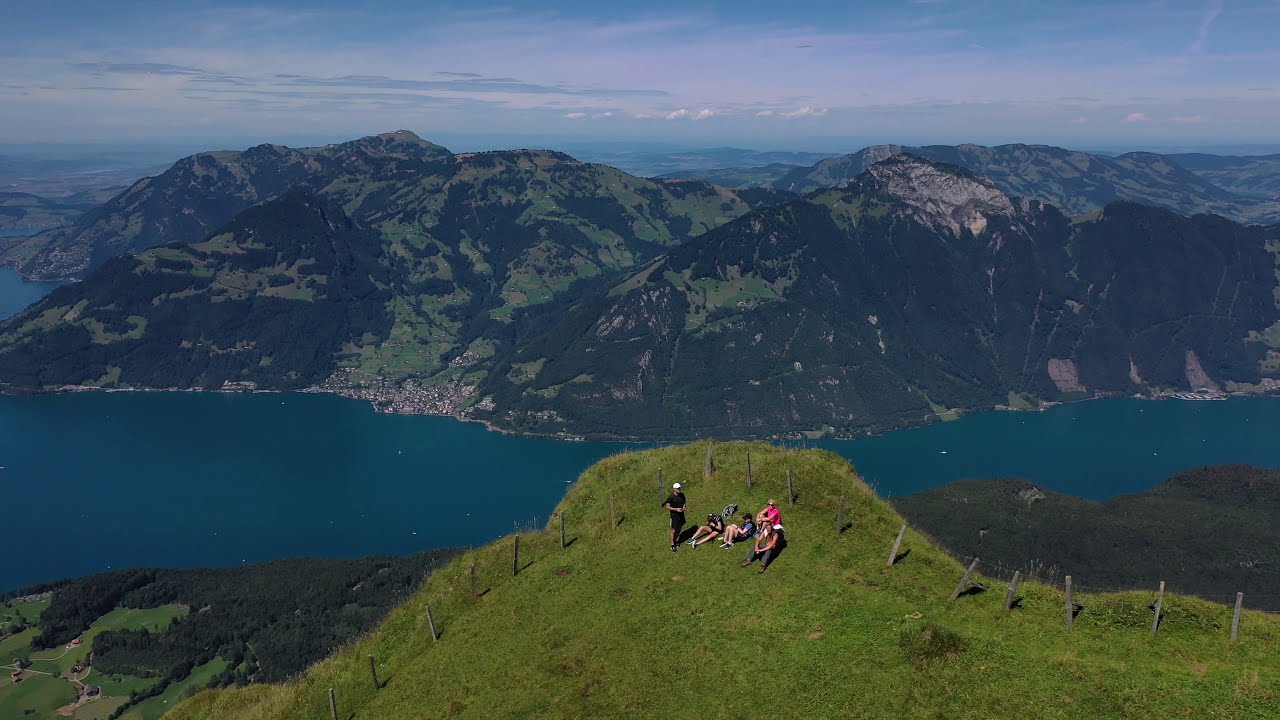In this high-altitude outdoor drone photograph, a vibrant, green hillside is the setting where a group of five people has gathered. Four sit with crossed legs near the edge, while one stands, operating a drone. He wears a white cap, dark blue t-shirt, jeans, and holds a drone controller, looking up at the device. A fence borders the cliff, providing safety. The scene overlooks a breathtaking deep blue lake nestled between two mountain ranges, with the far mountains framed by a serene sky dotted with a few clouds. On the lake’s shore, to the left, a small town and its buildings are also visible, highlighting the scale and elevated vantage point of this picturesque moment captured in vivid detail and striking realism.